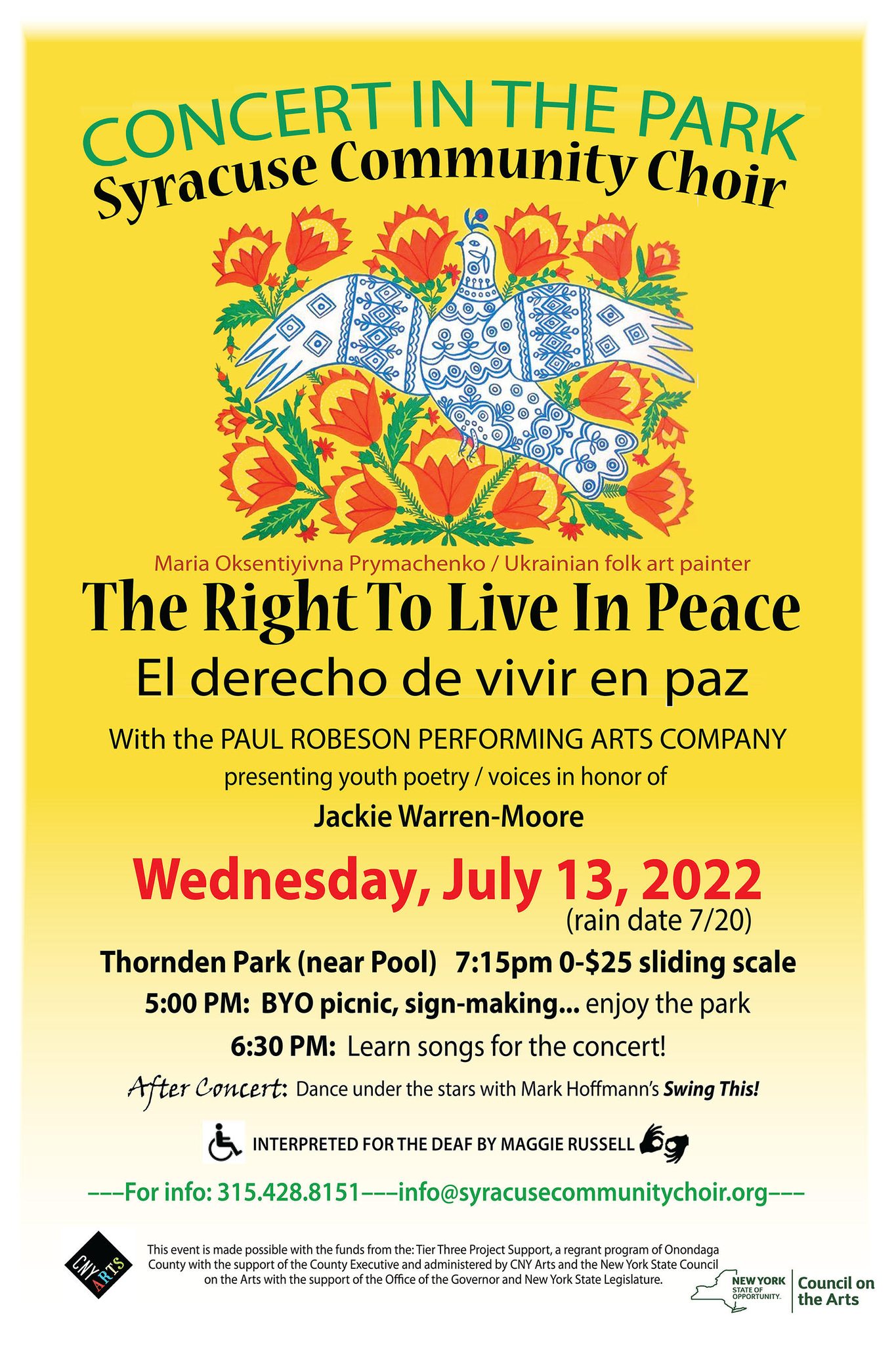The poster, set against a yellow background with striking green, black, blue, and red inks, advertises an event titled "Concert in the Park" featuring the Syracuse Community Choir. At the top, bold green text announces the event, while black text beneath recognizes the Syracuse Community Choir. Dominating the center is an illustration of a white bird adorned with blue tribal symbols, surrounded by vibrant red flowers and green leaves. Highlighted in large black text is the phrase "The Right to Live in Peace," alongside its Spanish translation, "El Derecho de Vivir en Paz." 

The poster indicates that the concert will take place on Wednesday, July 13th, 2022, at Thornden Park, near the pool, with a rain date on July 20th. Additional event details include a sliding scale admission of $0 to $25, beginning with a BYO Picnic Signmaking at 5:00 p.m., followed by song learning at 6:30 p.m., and the concert starting at 7:15 p.m. Post-concert festivities feature a "Dance Under the Stars" with Mark Hoffman's Swing This Band, interpreted for the deaf by Maggie Russell. The event is sponsored by the New York Council on the Arts and organized in collaboration with the Paul Robeson Performing Arts Company. For additional information, the poster provides a contact number, 315-428-8151.